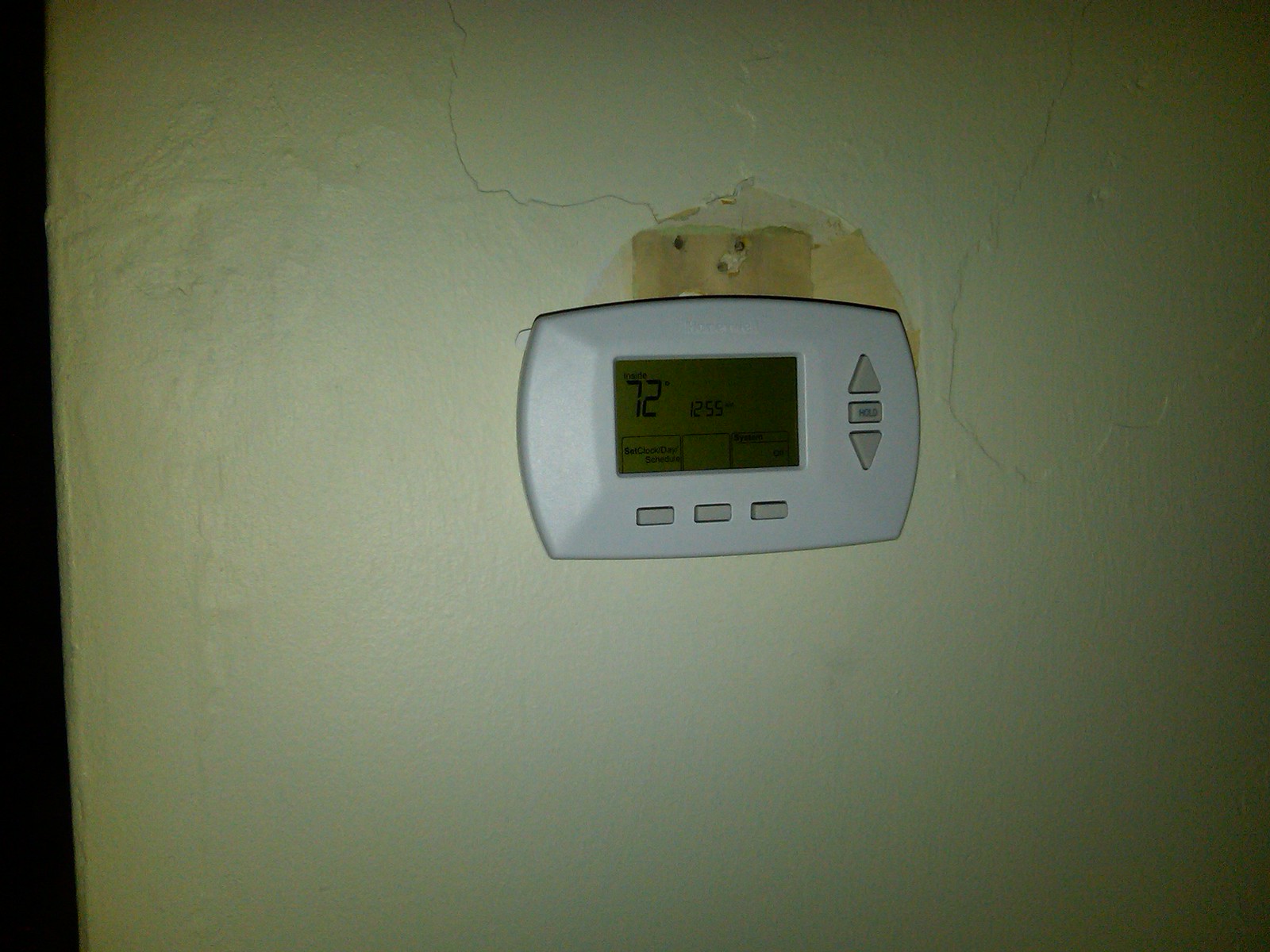This image showcases a white thermostat mounted on a white, stone wall. The thermostat has a slightly arched rectangular shape and is equipped with three buttons on the right side: an up button, a rectangular button labeled "Hold" in black text, and a down button. Below the screen of the thermostat, there are three gray rectangular buttons. The screen displays a temperature of 72 degrees Fahrenheit and the time as 12:55. Beneath the time display, three connected boxes are visible at the bottom of the screen.

Above the thermostat, there is an outline of what appears to have been an electrical outlet, identifiable by three screw holes at the top. The stone wall is marred by a significant crack that extends from the former outlet outline to the left and then upwards. The left side of the image is shrouded in darkness, highlighting the contrast between the illuminated thermostat and its surroundings.